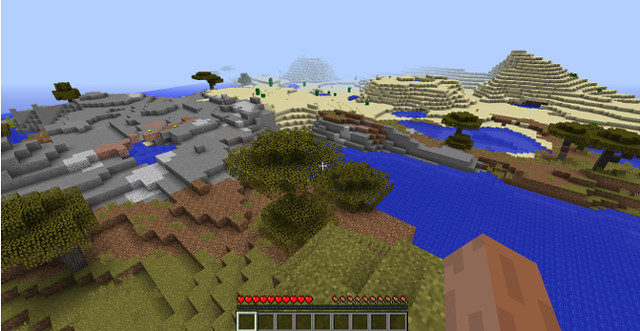The screenshot appears to be from Minecraft, featuring a player view with a distinctive blocky aesthetic characteristic of the game. In the foreground, the player's right hand is visible along with a HUD displaying nine dark green, empty inventory slots at the bottom of the screen. Above the inventory, there is a row of red hearts indicating the player's health. The player seems to be standing on a grassy hill made of green and brown cubes with a mixture of dead grass and a few scattered dead leaves.

In the middle distance, the terrain transitions into various elements: there are dirt cubes below on the hill, separated by patches of gray rock, and patches of sand dunes to the right. A pond or small bay intrudes into the landscape with blue water surrounded by land. Additionally, blocky trees stand around the landscape, characterizing the typical Minecraft environment. Overhead, a clear blue sky spans across the background, adding to the serene yet desolate appearance of the world.